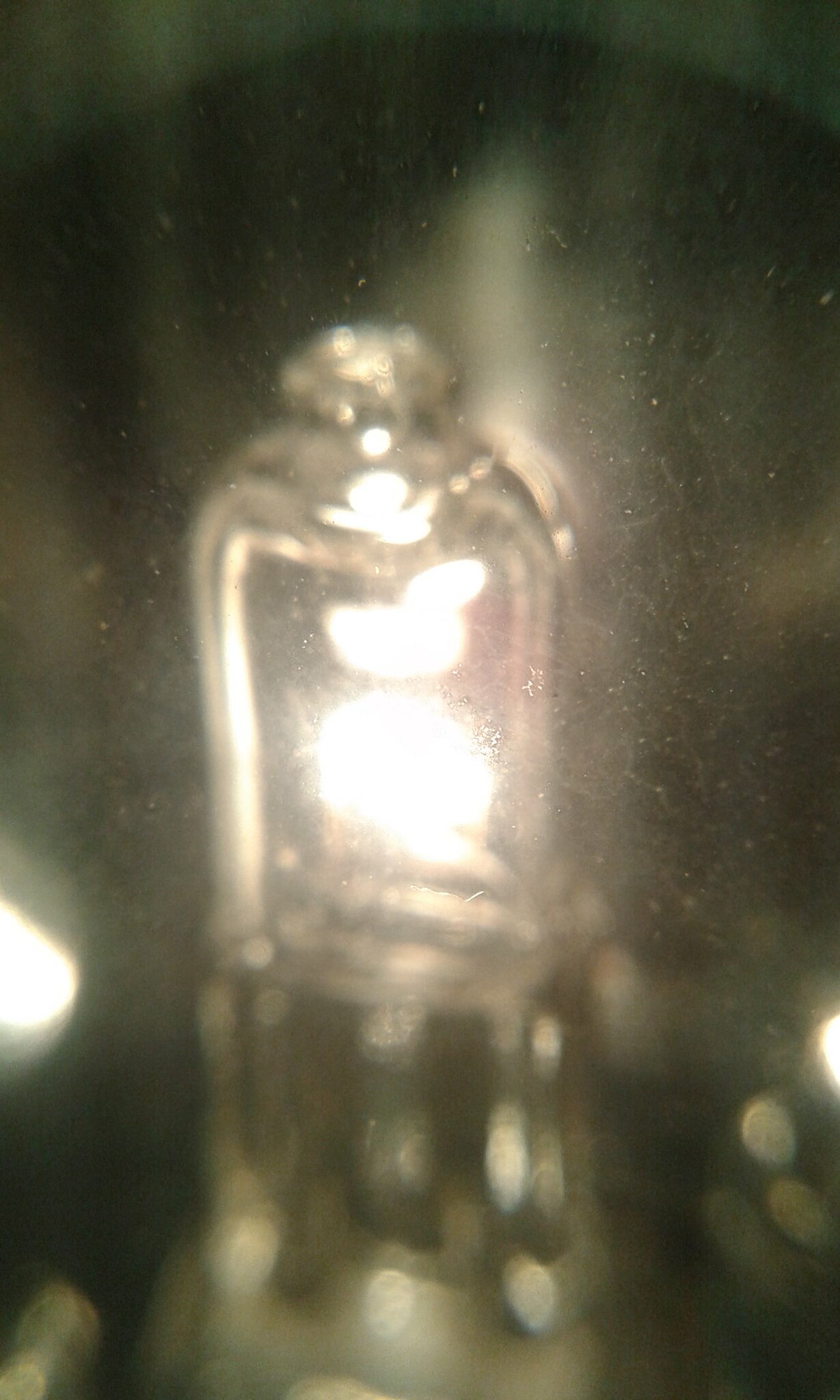This image is a very blurry photograph that portrays a light bulb-like object. The main focus is a glass or potentially plastic tube, somewhat rectangular with a round top, housing a glowing yellow filament. The image quality is poor, accentuated by various smudge marks which suggest it may have been taken through smudged glass. Below this main object, there appears to be a metallic or dark gray spherical base. Additional smaller, bright lights can be observed on the left and right sides of the image, though it's unclear if these are reflections or separate light sources. The background is predominantly dark gray and very indistinct, further contributing to the overall blurriness and white fuzz present throughout the photograph.